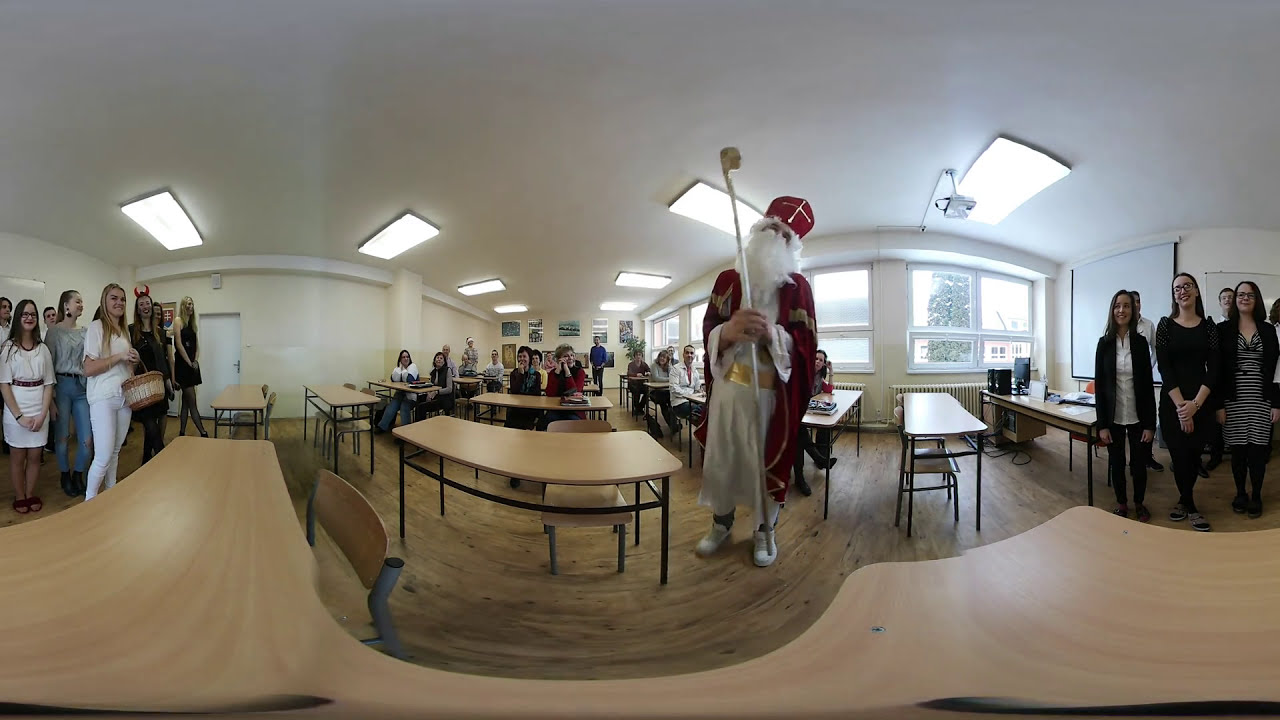The image captures a whimsical, indoor ceremony set in a white room with an eclectic mix of modern and vintage elements. The focal point is a person dressed in a St. Nicholas-like costume, featuring glowing, flowing red robes, a white garment, a gold belt, and a large red pope-like cap adorned with a cross. They hold a white staff and sport a full white beard, adding to the Santa Claus resemblance. Interestingly, they're also wearing modern sneakers, highlighting the ceremony's playful nature. 

The room is illuminated by large rectangular fluorescent lights on the ceiling, and there's an open window on the right side. The scene is filled with moderately young women dressed casually in dresses, pants, and blue jeans, all appearing to enjoy the light-hearted atmosphere as they smile and laugh. Several long tables are scattered throughout the room, surrounded by these participants.

The photograph is a composite panoramic image using a fisheye lens, consisting of three different vantage points: one showing a group of young women standing, another providing a straight-on view with people seated at tables, and the third giving a different angle of the same room. The dominant colors in the image are beige, black, white, tan, and gray, contributing to a casual, yet organized, classroom-like setting. The overall vibe suggests a less-than-serious, possibly humorous, gathering or event.